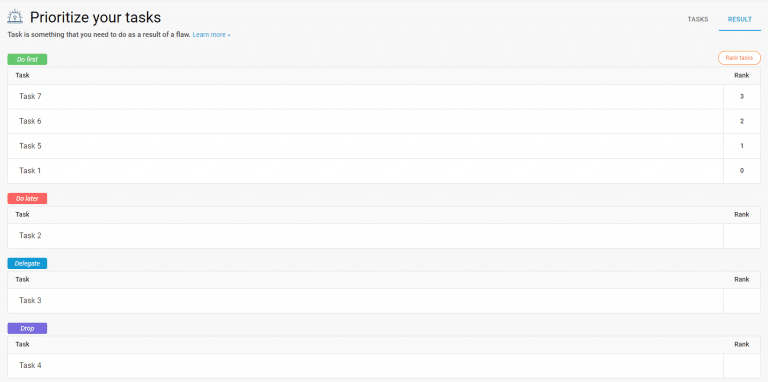**Detailed Caption:**

This image is a screenshot of a task management application with a light gray background. At the top left corner, the text "Prioritize Your Tasks" is prominently displayed. Below it, there's a blue "Learn more" link accompanied by a right-pointing arrow. On the top right, two options are available: "Tasks" in gray and "Result" in blue, with the latter underlined in blue.

The app is divided into four sections, each clearly delineated by colored labels and further organized into rows and columns. 

1. **Do First** - This section has a green label at the top left. Below the label, a gray bar lists two columns: "Task" and "Rank." The rows beneath this bar are white, separated by thin light gray lines, with tasks listed alongside their priority ranks. The tasks and their respective ranks are as follows:
   - Task 7, Rank 3
   - Task 6, Rank 2
   - Task 5, Rank 1
   - Task 1, Rank 0

2. **Do Later** - This section features a red label. It contains only one unranked task, named Task 2.

3. **Delegate** - Identified by a blue label, this section also includes a single unranked task, Task 3.

4. **Drop** - Marked with a purple label, this section has just one unranked task, Task 4.

The structured layout aids users in prioritizing and categorizing their tasks effectively.